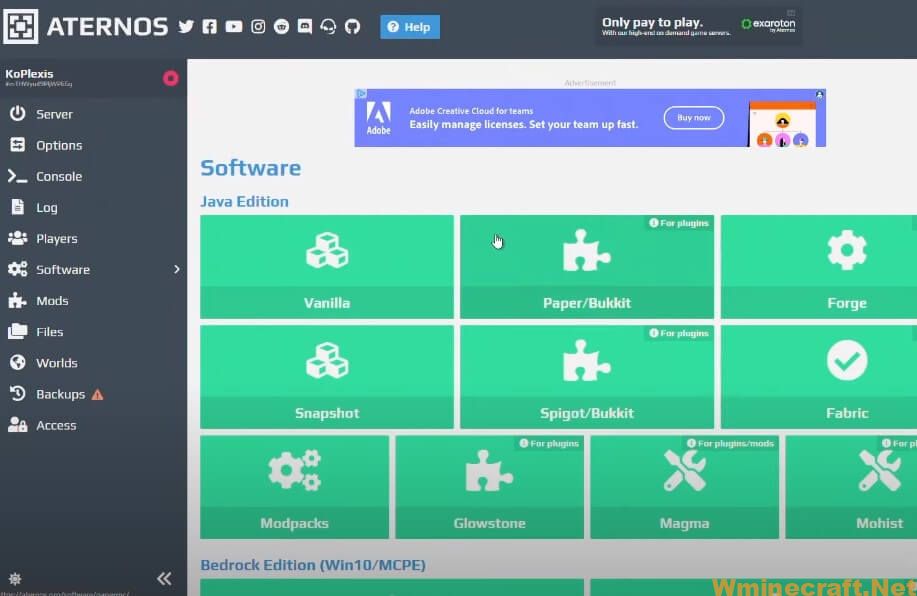The image is a detailed screenshot of the Aternos website, a platform known for providing free Minecraft server hosting. The layout features a distinctive design with a black-themed upper and lateral navigation bar, forming an upside-down 'L' shape. 

### Upper Navigation Bar:
- **Aternos Logo**: Positioned at the far left.
- **Social Media Icons**: Includes logos for Twitter (or its rebranded version), Facebook, YouTube, Instagram, Reddit, and several lesser-known platforms.

### Right Section of the Bar:
- "Only pay to play" is prominently displayed.

### Left Vertical Side Panel:
- **CoPlexus**: Displayed at the top as a section.
- **Record Button**: Represented by a red button with a black square in the center.
- **Power Switch Icon**: Labeled "Server," commonly referred to as the on-off switch.
- **Options Icon**: Depicted by a dial, with the word "Options" next to it.
- **Console**: Marked by a greater-than sign followed by an underscore.
- **Log**: Illustrated by an icon of flipping paper.
- **Players**: Represented by a standard group icon.
- **Software**: Signified by a cog with two circles extending from it.
- **Mods**: Indicated by a puzzle piece.
- **Files**: Displayed with a folder icon, followed by subcategories: "Worlds," "Backups," and "Access."

Overall, the image provides a comprehensive look at the Aternos website's user interface, illustrating various navigation options and functionality available for managing Minecraft servers.